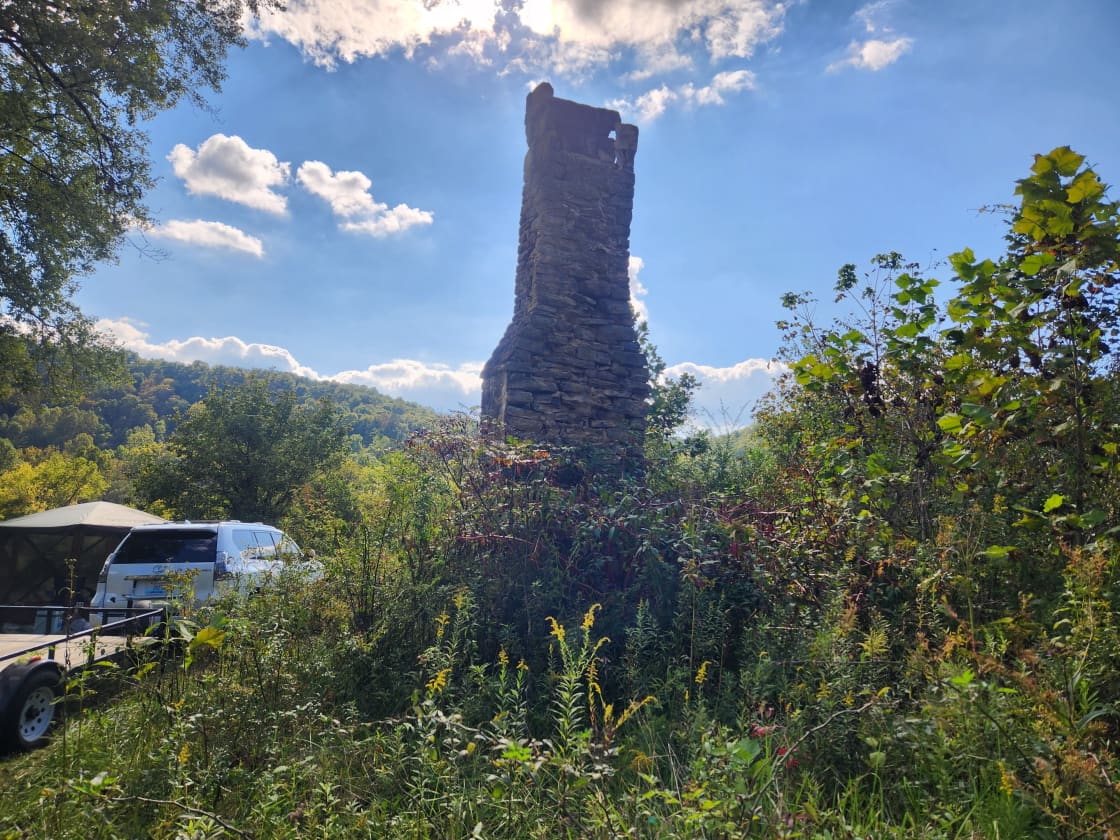The photograph captures a serene, sunlit wilderness scene, with the remnants of a once-standing cabin dominating the foreground; only a tall, rock chimney remains amidst a dense tangle of weeds, briars, and scattered shrubs, some adorned with little flowers, others showing the beginnings of trees. To the left, an SUV pulling a trailer is parked near a small roofed picnic area, potentially occupied. Beyond them, a ridge gently descends into a heavily forested valley, providing a lush, green backdrop that complements the clear blue sky dotted with a few bright white clouds, indicative of a warm midsummer or late spring day. A light-colored station wagon is also visible, suggesting the presence of campers perhaps enjoying the picturesque, mountainous landscape that could be found in locales like North Georgia, Northern Alabama, or the Virginias.